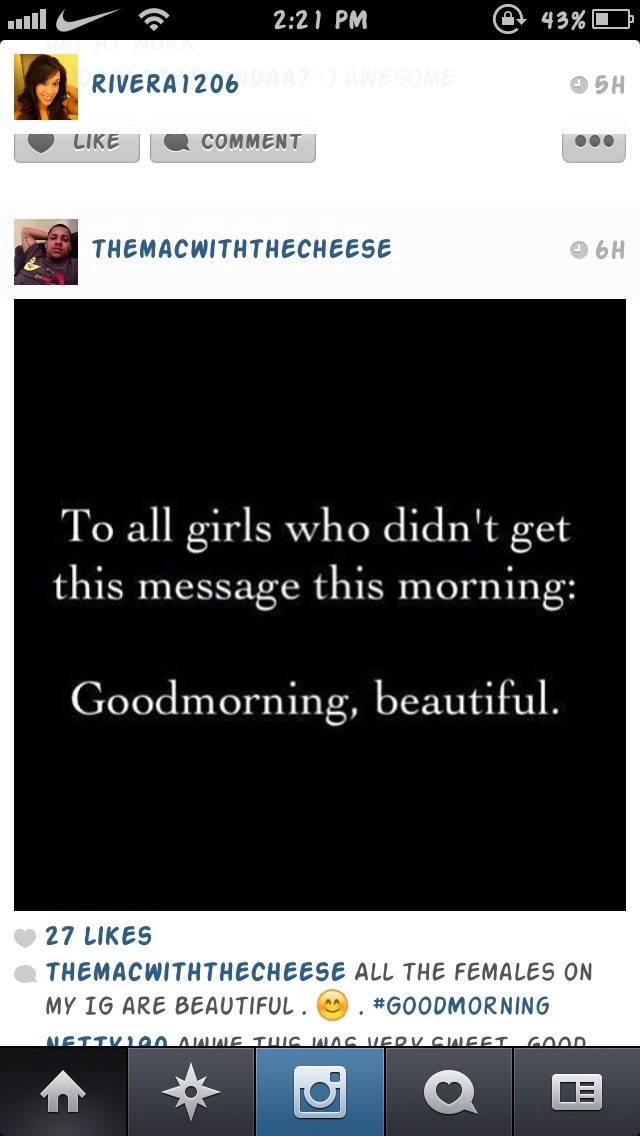This image depicts a smartphone screenshot from Instagram, evident from interface elements such as the signal bars, Wi-Fi logo, time (2:21 PM), and battery level (43%) at the top. The post is by a user named "The Mac with the Cheese," who appears to be a young man with short-cropped hair, posing with one hand behind his head. The screenshot was taken by another user, "Rivera 1206," a young woman with long black hair. The central content of the image is a black background with white text that reads, "To all girls who didn't get this message this morning, good morning beautiful." The post has 27 likes and a comment from "The Mac with the Cheese" saying, "All the females on my IG are beautiful," followed by a smiley face emoji and the hashtag #goodmorning. The bottom of the screen shows Instagram icons, suggesting it's a meme or motivational message shared on social media.